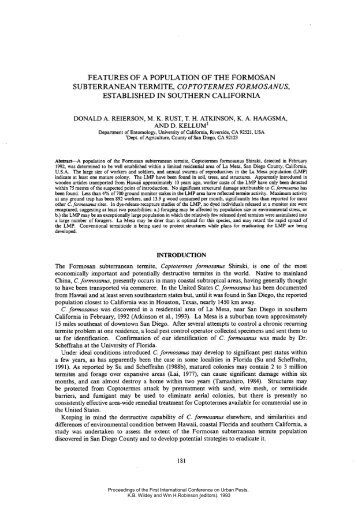This image depicts a page from a scientific journal, specifically page 181. The title at the top reads "Features of a Population of the Formosan Subterranean Termite, Coptotermes formosanus, Established in Southern California," emphasizing an invasive species. Directly beneath the title, smaller text lists the authors: Donald A. Riverson, M. K. Rust, T. H. Atkinson, K. H. Hagsma, and D. Kellum. This is followed by a paragraph providing further details, although the print is too small to make out precisely. The bold heading "Introduction" is clearly visible, followed by four paragraphs of indistinguishable text. The visual layout and structure suggest this is a detailed article possibly discussing the ecological and economic impacts of the Formosan subterranean termite in Southern California.